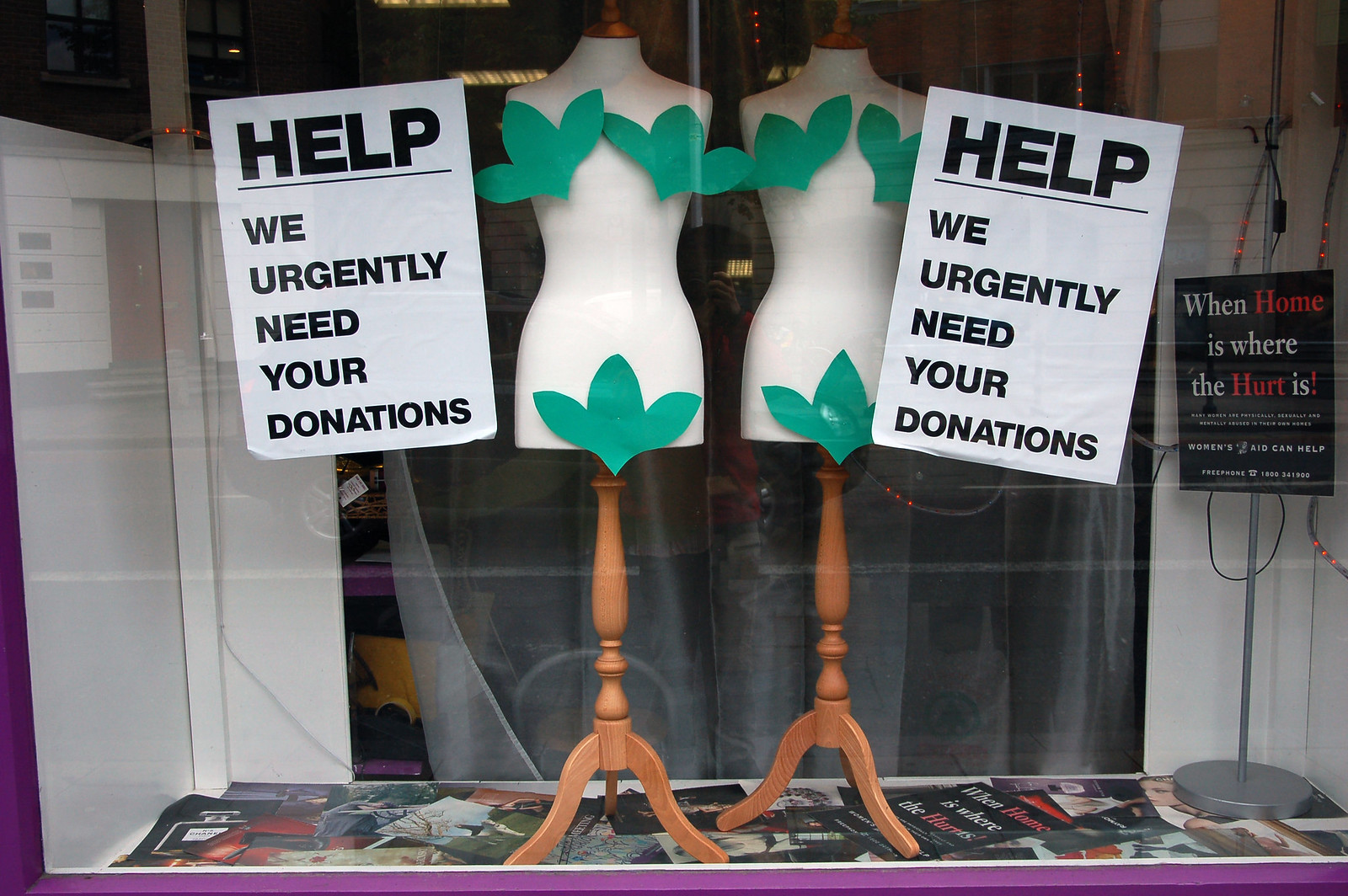This photograph, taken in landscape orientation through the window of a department store, reveals a poignant display. At the center are two white, female torso mannequins adorned with hand-cut leaves covering their breast and groin areas, mounted on a wooden stand. Flanking the mannequins on either side are two large flyers that read, "Help, we urgently need your donations." To the right, a black sign on a metal pole stands out with red and white text, "When home is where the hurt is," and further below, "Women's aid can help." Scattered beneath the mannequins are similar flyers. The backdrop includes a gray, semi-transparent curtain, partially peeled back at the left corner, revealing indistinct devices and objects in the background.